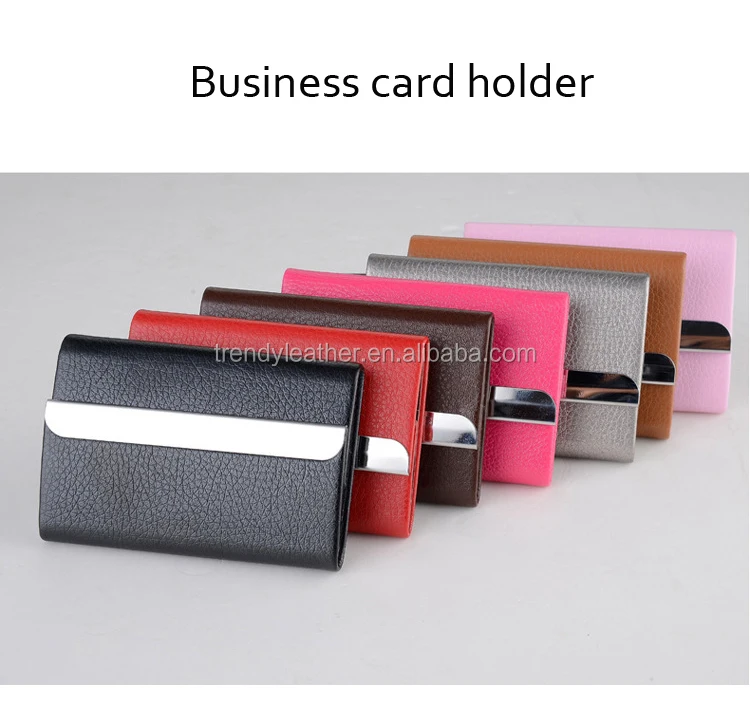The image, possibly from an advertisement or online catalog, features a collection of seven business card holders arranged against an off-white background. The top of the graphic displays the text "Business Card Holder" in black on a white background. The business card holders, which appear to be made of either real or synthetic leather, come in a variety of colors: black, red, dark brown, pink, gray, light brown, and light pink. Each holder is adorned with a silver metal accent piece on the front. Across the center of the image, in light gray text, is the website "trendyleather.en.alibaba.com."